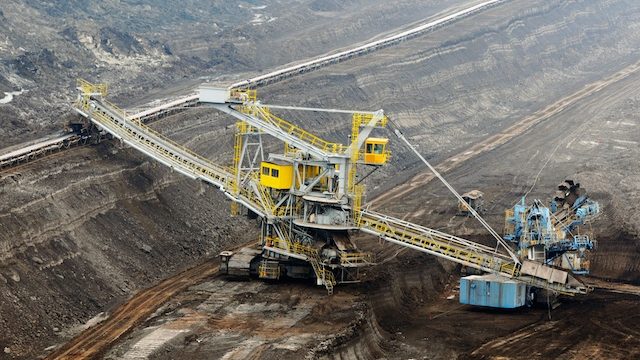The image depicts an expansive, barren rock quarry taken from a high vantage point during the daytime. Dominating the scene is a massive, brightly-colored yellow crane or excavator, distinguished by its tank-like treads at the base and multiple levels accessible via staircases and ladders. The crane's center cabin is a focal point, with additional cockpits atop the machinery. Long excavation arms, reminiscent of conveyor belts, extend from the machinery, indicating active work. To the right, there are several metal containers, including a noticeable blue rectangular one, adding to the industrial ambiance. The ground is a stark, dark brown and gray, devoid of vegetation, and channels are dug into it, possibly with rails installed in the upper left section. Further in the background, a small shed stands alone, emphasizing the emptiness of the field that is intersected by patches of dirt and sparse grass. The air appears hazy in the distance, casting a somber mood over the quarry, with the bright yellow crane serving as the only vivid element in an otherwise muted, desolate landscape.